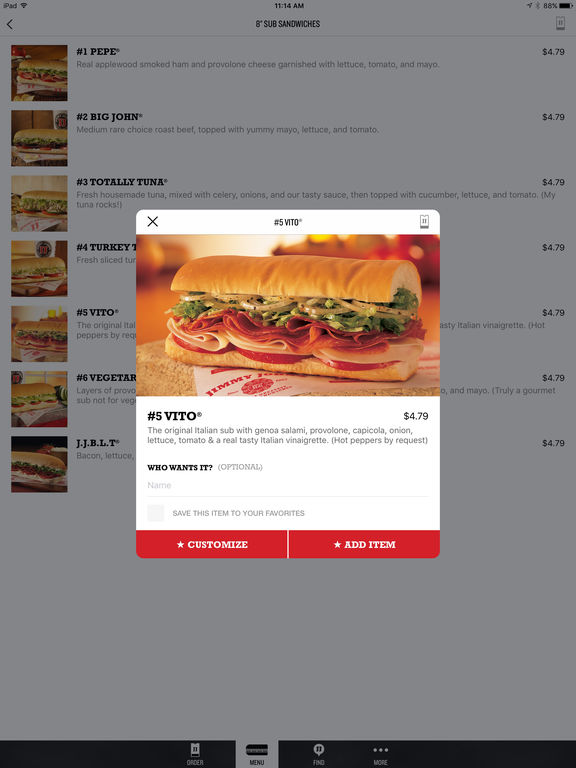**Detailed Descriptive Caption:**

This screenshot, captured from an iPad interface, displays a menu list for 8-inch sub sandwiches.

In the top-left corner, it shows the text "iPad" along with the Wi-Fi symbol. Centrally at the top, the time is displayed as "11:14 AM". On the top-right corner, there is a navigation symbol, a Bluetooth indicator, and the battery icon which indicates 88% battery remaining.

Below the time display, centered, the screen shows "8 INCH SUB SANDWICHES" in all caps. On the left side, below the Wi-Fi symbol, there is an arrow pointing to the left, while the right side, below the battery indicator, features a ticket symbol.

The detailed listings for the sub sandwiches begin with the first option:

1. **#1 Pepe**  
    - Image of the sandwich.
    - Ingredients: Real Applewood smoked ham and provolone cheese garnished with lettuce, tomato, and mayo.
    - Price: $4.79.
    
2. **#2 Big John**  
    - Image of the sandwich.
    - Ingredients: Medium rare choice roast beef topped with yummy mayo, lettuce, and tomato.
    - Price: $4.79.

3. **#3 Totally Tuna**  
    - Image of the sandwich.
    - Ingredients: Fresh homemade tuna mixed with celery, onions, and their tasty sauce, topped with cucumber, lettuce, and tomato (My tuna rocks!).
    - Price: $4.79.

4. **#4 Turkey Tom**  
    - Image of the sandwich.
    - Ingredients: Fresh sliced turkey breast.
    - Price: $4.79.

5. **#5 Vito**  
    - Image of the sandwich.
    - Ingredients: The original Italian sub with genoa salami, provolone, capicola, onion, lettuce, tomato, and a real tasty Italian vinaigrette (Hot peppers by request).
    - Price: $4.79.
    - Below the ingredients: "Who wants it?" with an optional checkbox to associate this item to your favorites.

6. **#6 Vegetarian**  
    - Image of the sandwich.
    - Ingredients: Layers of provolone cheese separate avocado, sliced cucumber, lettuce, tomato, and mayo (Truly a gourmet sub for veggie lovers).
    - Price: $4.79.

7. **JJBLT**  
    - Image of the sandwich.
    - Ingredients: Bacon, lettuce, tomato, and mayo.
    - Price: $4.79.

At the bottom of the screen, a black bar contains several controls. It shows a ticket icon with the text "Order" next to it, followed by an icon of a sandwich with "Menu" underneath, a communication symbol with "Find" below it, and three dots labeled "More".

Buttons at the bottom of some of the listings, within a red box, include "Customize" on the left and "Add Item" on the right, in white text.

This detailed menu layout is designed for a convenient browsing and ordering experience on the iPad.